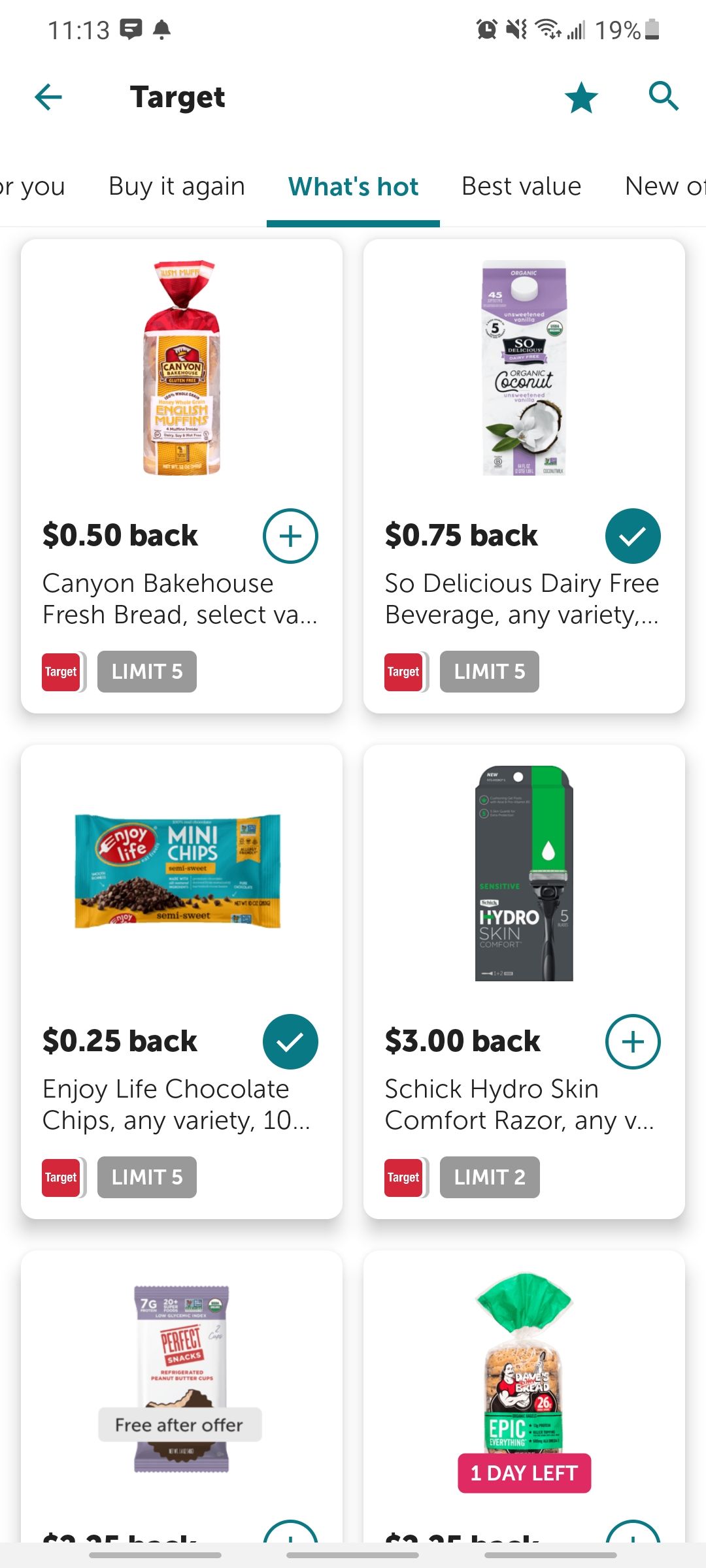This screenshot depicts a smartphone screen displaying the Target mobile app on an Android device. The phone shows typical mobile interface elements, including a 90% battery level, an alarm set, muted ringer, and the current time of 11:13 AM. Various notifications, including text messages, can be seen.

The Target app is open in light mode and is currently showcasing the "What's Hot" section. The screen presents several categories such as "For You," "Buy It Again," "Best Value," "New Items," and "New Orders." At the top right corner, there is a clickable star button, presumably for favoriting items, next to a magnifying glass icon used for searching products within the app.

Highlighted deals include:
- A loaf of bread with a 50 cent cashback.
- Coconut milk with a 75 cent cashback.
- Mini chips with a 25 cent cashback.
- Schick Hydroskin Comfort razors offering 3 dollars back.
Additional items displayed feature more bread on the right side and chocolate on the left side of the screen.

The detailed layout and elements indicate the user is browsing through various cashback offers on grocery and personal care items.